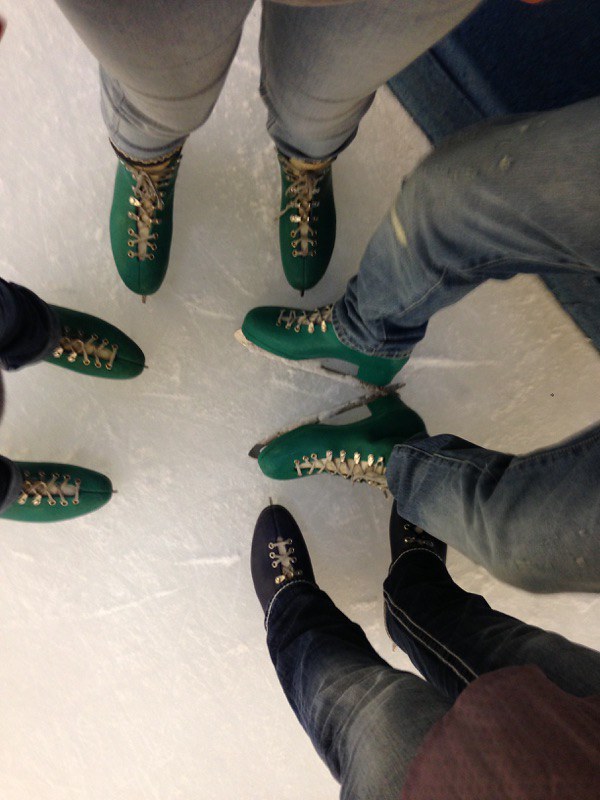This aerial photograph portrays a cluster of four individuals at an ice skating rink, their feet and legs central to the composition. The group stands on a light gray and white ice surface, marked with striations from skating. Three of the individuals wear green ice skates with gold laces, while the fourth person sports black skates with black laces. Their attire includes various shades of jeans—medium blue, gray, and black. One person in black jeans and a burgundy hoodie appears to be sitting on a navy blue seating visible in the upper right corner, suggesting a casual moment next to the bench. The image exudes a sense of camaraderie and shared experience, likely captured to commemorate a fun outing together.